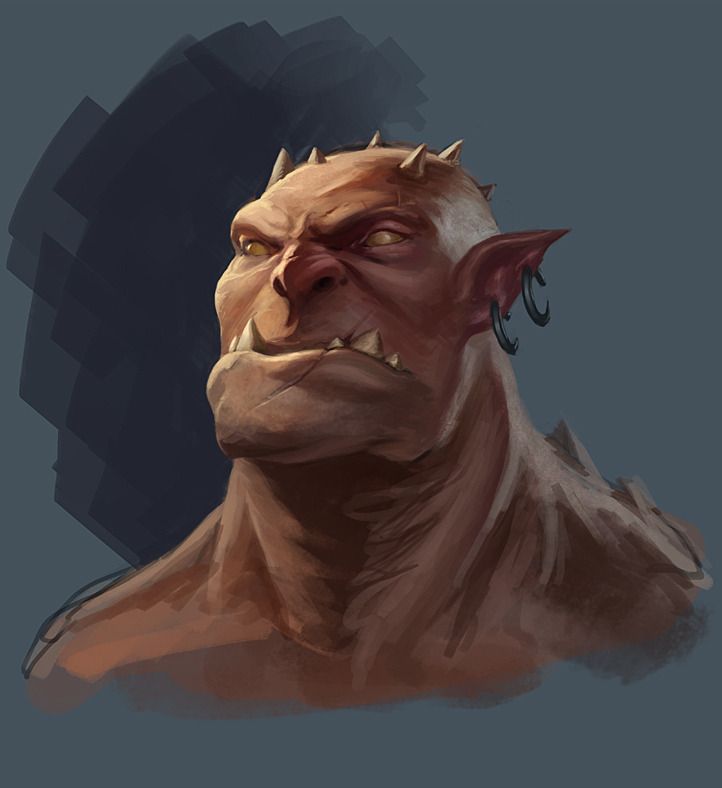The image is a screenshot from the website PhotoBucket, captioned with the tagline "Protect More of Your Memories for Less" on a white strip. The photograph shows a square depiction of a monstrous creature from the shoulders up against a dark navy background. The creature has a bald, pinkish, leathery flesh tone that resembles a human man. Its head is adorned with six thick, bone-colored spikes that resemble horns. The creature's eyes are hollow and goldish, appearing almost inhuman. It has large, pointed ears with two black hoops pierced through one of them. Its nose is big with flaring nostrils, and its mouth features an underbite with jagged, protruding teeth that are shaped similarly to the spikes on its head.